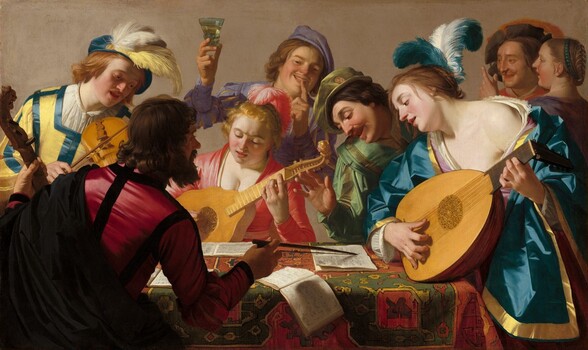In this Renaissance-era oil painting, a lively group of musicians is gathered around a richly adorned table, engrossed in a music manuscript. At the center, a bearded man with long brown hair, dressed in a red long-sleeved shirt and draped with a black cloth, sits at the table. He points to the music notes with a wooden pointer, likely indicating his role as a composer or conductor. The table itself boasts a lavish red and green patterned tablecloth, and an open book precariously hangs off its edge.

To the composer's left, a woman in a lavish green and gold cloak, draped stylishly off her shoulder, strums a round guitar-like instrument. Her hair is elegantly pulled back, adorned with matching feathers. Directly across from her sits another woman, highlighted by a light focusing on her décolletage. She has red hair, accented by pink feathers, and wears a coral-pink garment while playing a gourd-shaped string instrument, possibly a lute.

Standing near the composer, a man in a green outfit studies the music sheet closely, raising his hand in thought. Behind him, a youth dressed in a purple outfit and cap jovially lifts a glass of spirits, a mischievous finger to his lips. In the background, another couple appears engaged and smiling, absorbed in their own conversation.

On the upper left side of the painting, a boy with long red hair is engrossed in playing a violin. He sports a yellow jacket with teal ribbons and a white tunic, with a feathered cap completing his colorful attire. The backdrop of the painting features muted brown walls, adding to the intimate, vintage ambiance of the scene.